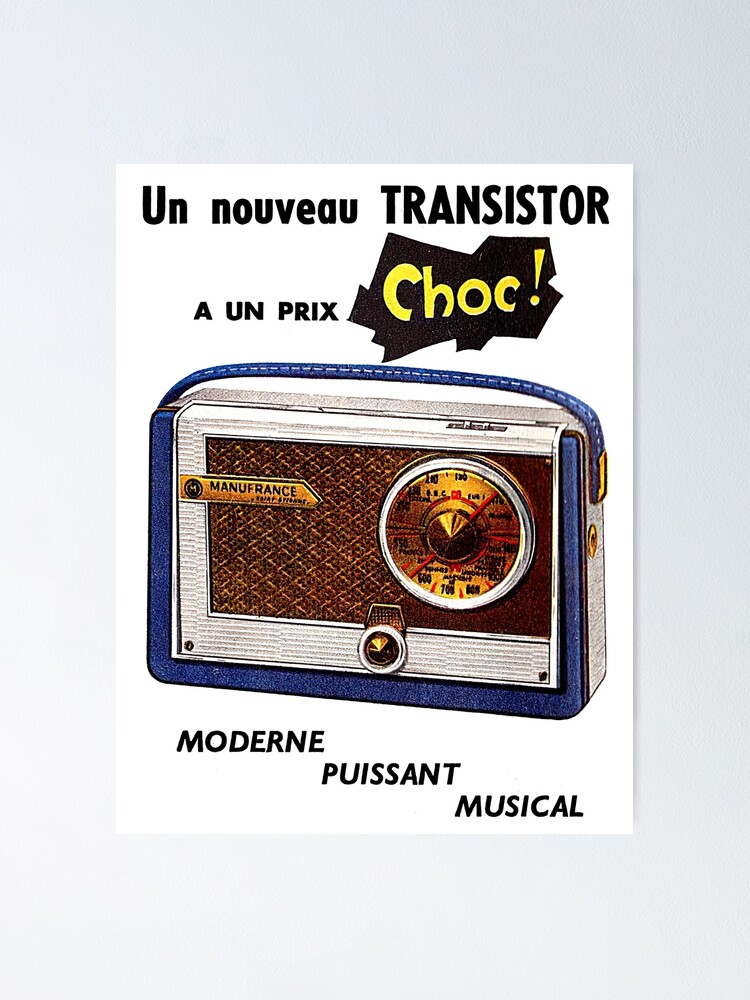This image is a detailed French advertisement for a vintage radio designed to resemble a purse. The text on the ad reads "Un Nouveau Transistor à Un Prix Choc," promoting an affordable new transistor radio, and "Moderne Façon Musical," highlighting its modern, musical styling. The radio itself is a blend of several materials and colors: it features a blue and white trim with a blue handle, making it portable and stylish. It has a brass front panel with a knob tuner, marked by a red line indicating the tuned station. The brand "Manufrance" is displayed on the left side of the radio's face, identifying its French origin. The radio is further detailed with a gold latch connecting a cloth strap, enhancing its purse-like appearance. A gold circle on the right denotes a headphone jack set against the grey cloth background, while speaker grills wrap around the brass front. The soft cloth finish adds to its portability, suggesting compartments at the top for additional functionalities such as input or tape insertion. This meticulously designed radio merges fashion with functionality, making it a unique piece of audio equipment.